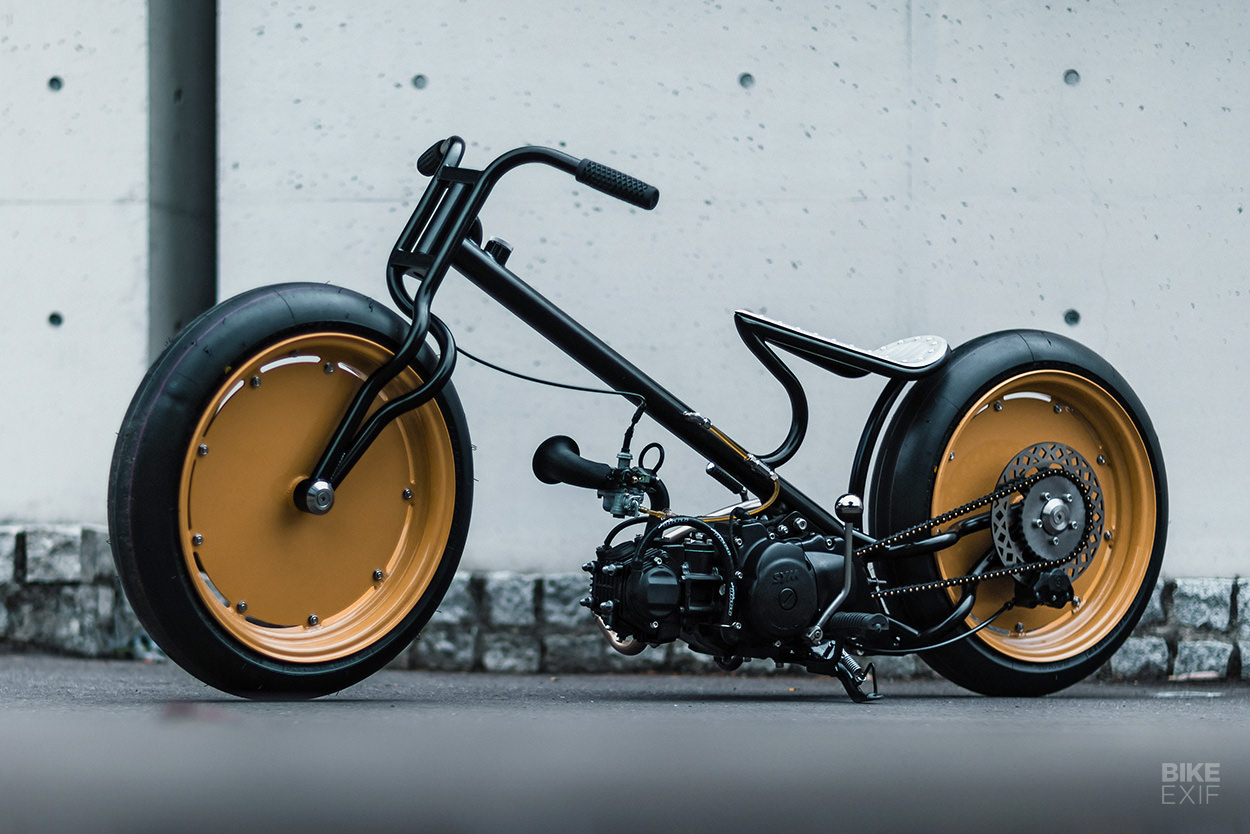The image features a unique and simplistic motorized bike, primarily black with notable design elements. The large, bronze-colored wheels and black tires stand out, with the rims being described as either yellow or golden brown. The handlebars extend unusually low, almost touching the ground, giving the bike a distinctive appearance. The bike's frame is black, and it includes a banana seat, but there's no visible gas tank, suggesting it might be an electric bike or a pedal-assist model. The motor is positioned unusually low, almost touching the ground. The background is a faded black and white scene that includes a short brick wall, a fence, and the sky, with the bike itself in vivid color. The ground is cement, and there are visible holes in the cement tiles. A watermark reading "BIKE EXIF" is located in the bottom right corner of the image.